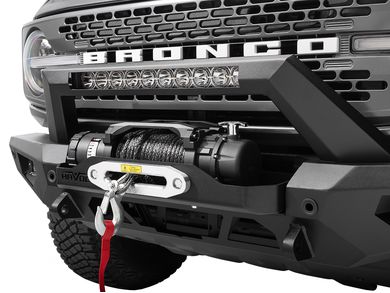This photograph showcases the front of a brand new Ford Bronco, emphasizing its off-roading capabilities. The truck, appearing to be black or dark gray, features a prominent black grille marked with the word "BRONCO" in bold white letters. The grille is designed with an array of consecutive rectangular holes, ensuring airflow to the radiator. The vehicle is equipped with several off-roading accessories, including a heavy-duty towing winch attached to the front bumper. This winch features a robust cable wound around a reel, ending in a silver hook with a red tag for safety. A light bar and additional lights positioned on the bumper enhance the truck's rugged aesthetic and functionality. Part of a round headlight is visible, indicating the vehicle is likely not in use as the headlights are off. The bumper houses multiple lights, further preparing the Bronco for off-road adventures. The overall condition of the vehicle suggests it is brand new, free of scratches or dents, with its tough design and bulky tires ready for mud and off-road challenges.